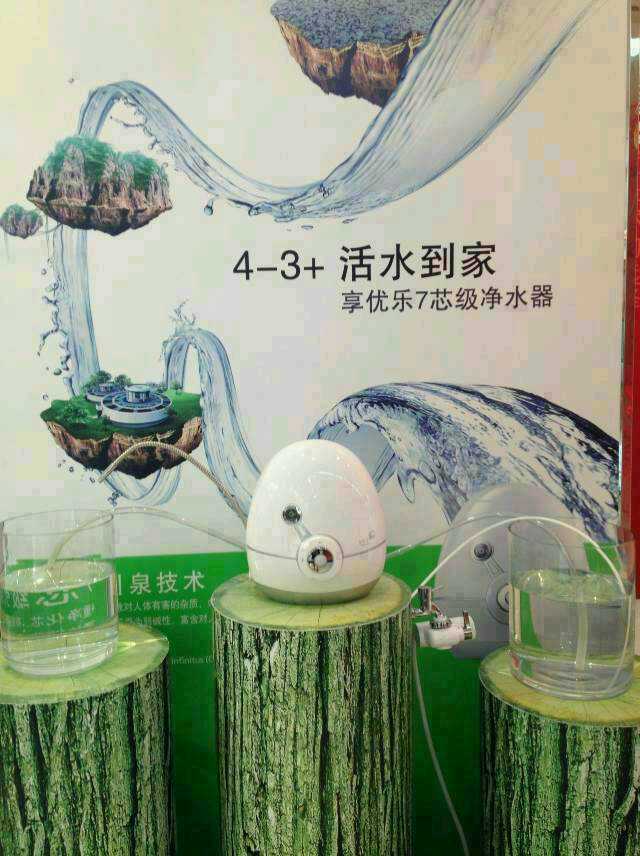In the image, there is a detailed experimental setup featuring three green log-like tables, clearly artificial in nature. At the center of these tables sits an oversized, egg-shaped white device, with clear hoses extending from it to substantial glass containers of water positioned on the adjacent logs. The backdrop of the scene is a large, white poster depicting a whimsical landscape of floating islands and flowing water, starting from a mountain on the top left and meandering down to a grassy platform at the bottom left. Embedded in this fantastical terrain are gray clouds and possibly circular houses perched on the sliced stumps of jagged trees. The poster includes an assortment of Asian characters and the equation "4 - 3 +" prominently placed next to the text, suggesting the setting is an advertisement or educational display from an Asian country. The detailed combination of the setup and visually rich background hints at a possible water filtration demonstration or conceptual art piece.